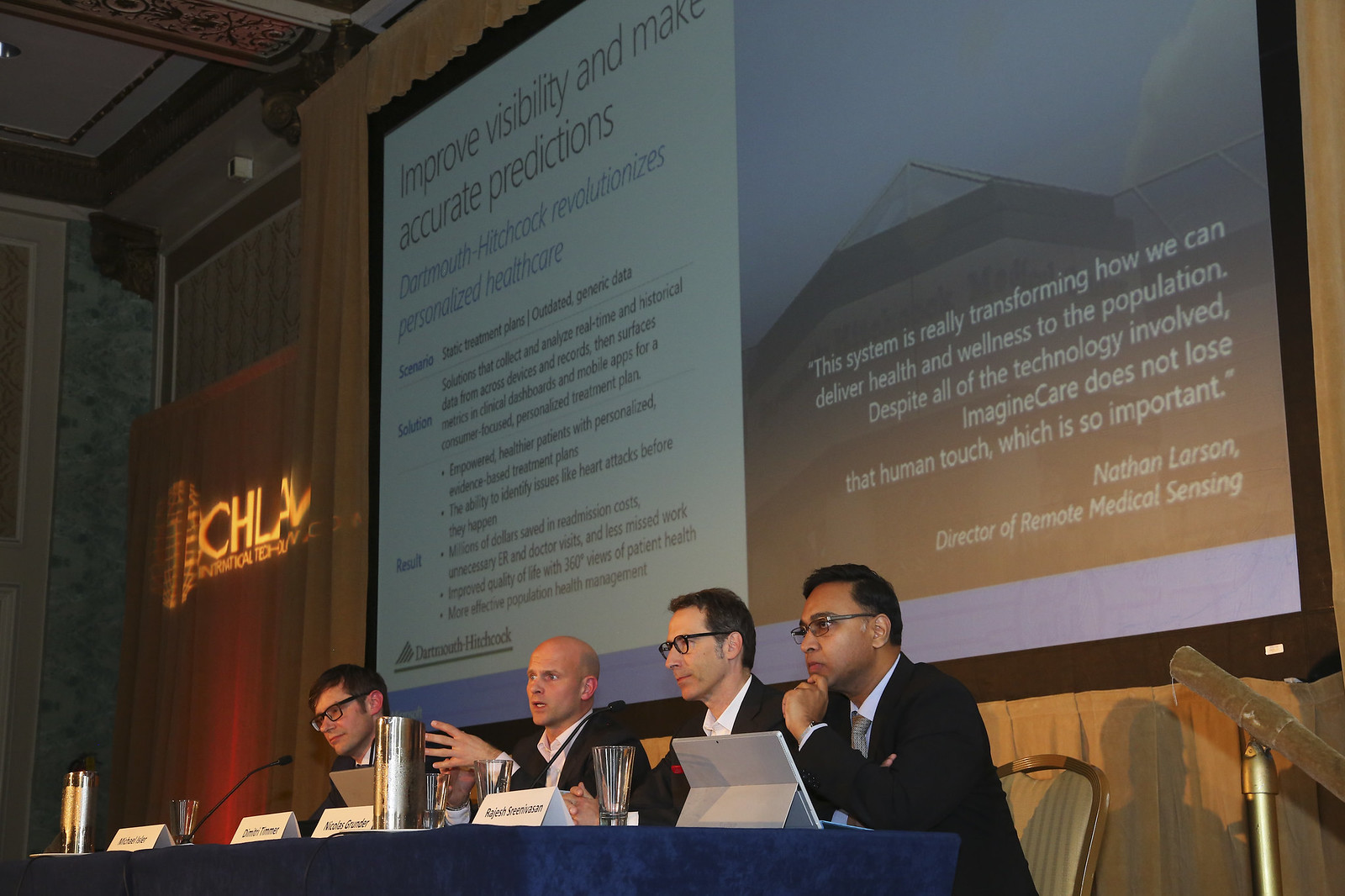This image captures a panel of four men seated behind a blue-covered podium during a conference set in an auditorium or hall. Each man is identified with a name tag: from left to right, Michael Eisler, Dimitri Trimmer, Nicholas Groomer, and Rajesh Srinivasan. The men are dressed in black suits and wear glasses, except for one who is bald and not wearing specs. In front of them are empty water glasses, a metallic pitcher, microphones, and open laptops or iPads.

Behind the panel, a large flat projector screen with black borders displays a detailed slide with several key messages about improving visibility and making accurate predictions in personalized healthcare, led by Dartmouth-Hitchcock. The highlighted points on the screen include the importance of real-time and historical data analysis to create personalized, evidence-based treatment plans, ultimately resulting in empowered patients, improved quality of life, and significant healthcare cost savings. The screen also features a quote from Nathan Larson, Director of Remote Medical Sensing, emphasizing the balance of technology and human touch in transforming healthcare delivery.

The backdrop of the room includes a brown wooden wall, a ceiling with visible fixtures, a door with a red banner bearing partially legible text and logos, and a CCTV camera. The comprehensive setting suggests a formal, informative conference aiming to discuss advancements in personalized healthcare.